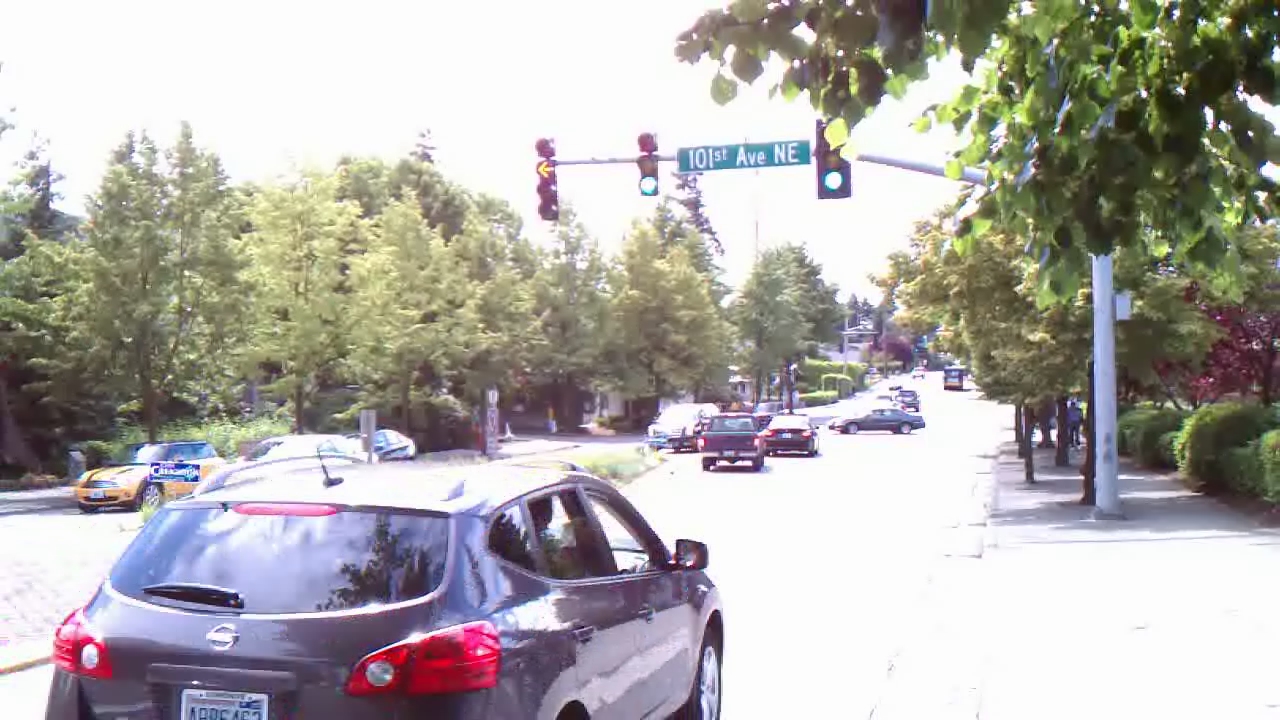Under a bright, luminescent white sky, the scene below is partially illuminated, casting a gentle light on the ground. The left side is adorned with numerous trees, their leaves a soft, light green hue. In contrast, the right side features trees with larger leaves, including one remarkable tree with striking purple foliage. A gray sidewalk winds through the scene, accompanied by a street post. Above, three traffic lights are prominently displayed, with a sign indicating the intersection of 101st Avenue and 8th Street. The traffic lights show a green light both on the left and the right, and a white pedestrian signal can be seen as well. A yellow arrow points left, nestled among clusters of green leaves in the middle of the scene. Below, a sleek black compact car with visible windows stands near the foreground, while more cars, hinting at active traffic, are visible in the distance. On the left, a vibrant yellow sports car with striking black stripes adds a flash of color to this dynamic streetscape.